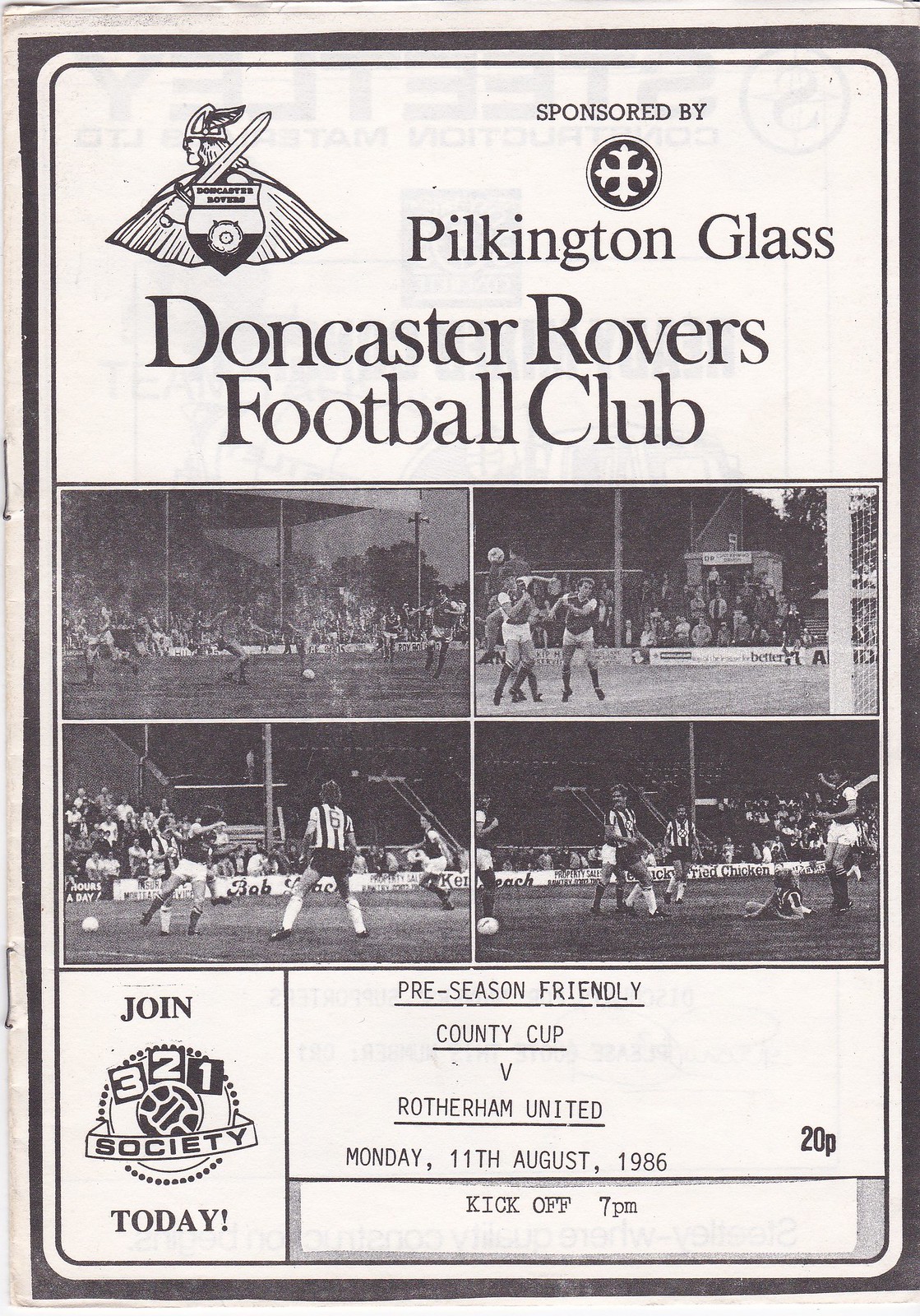This is a scanned black-and-white pamphlet, likely a program or advertisement, for the Doncaster Rovers Football Club, sponsored by Pilkington Glass. The pamphlet features a dark gray background with gray and white text. At the top, the club's insignia depicts a warrior with a feather in their headgear, wielding a sword and shield. Below this are four black-and-white photos forming a collage of soccer games, showcasing players in action, referees in black and white striped shirts, and spectators in the stands. The players are dressed in distinctive uniforms, with some wearing dark shirts and others in lighter shirts, typical long socks, and short shorts. The pamphlet announces a preseason friendly County Cup match against Rotherham United, scheduled for Monday, 11th August 1986, with a kickoff at 7 p.m. Additionally, it invites readers to "join the 3-2-1 society today."